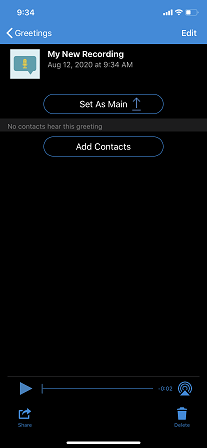This image is a screenshot from a smartphone, containing various interface elements. The top banner is blue with a timestamp of 9:34 in white text on the left. On the right, it displays icons for cell service (represented by footballs), Wi-Fi signal strength, and a battery indicator showing around 50% charge.

Below the top banner, the screen has a header with "Greetings" in bold white text followed by a left-facing arrow on the left, and "Edit" on the right. The main part of the screen has a black background.

At the top of the black screen, the text "My New Recording" appears in bold white print, followed by the date "August 12th, 2020 at 9:34 A.M.". To the left of these details, there is a white square housing a blue sound wave icon with a yellow microphone inside it.

Further down, a white text label says "Set as Main," enclosed within a blue-bordered, rounded rectangle resembling a hot dog. Below this element is a blue upward-pointing arrow with a line beneath it.

A lighter black, grayed-out banner follows, containing the text "No Contacts Here This Greeting" in white. Directly below this, there is another white text label "Add Contacts," again within a blue-bordered, rounded rectangle.

The bottom portion of the screen is primarily black, but at the very bottom, there are several icons and text elements. On the left, there is a blue sideways triangle pointing towards the right. Below this, the word "Share" appears alongside a rectangle with an arrow protruding from it. There is also a timestamp reading "-0:02" and a "Delete" option with a trash can icon.